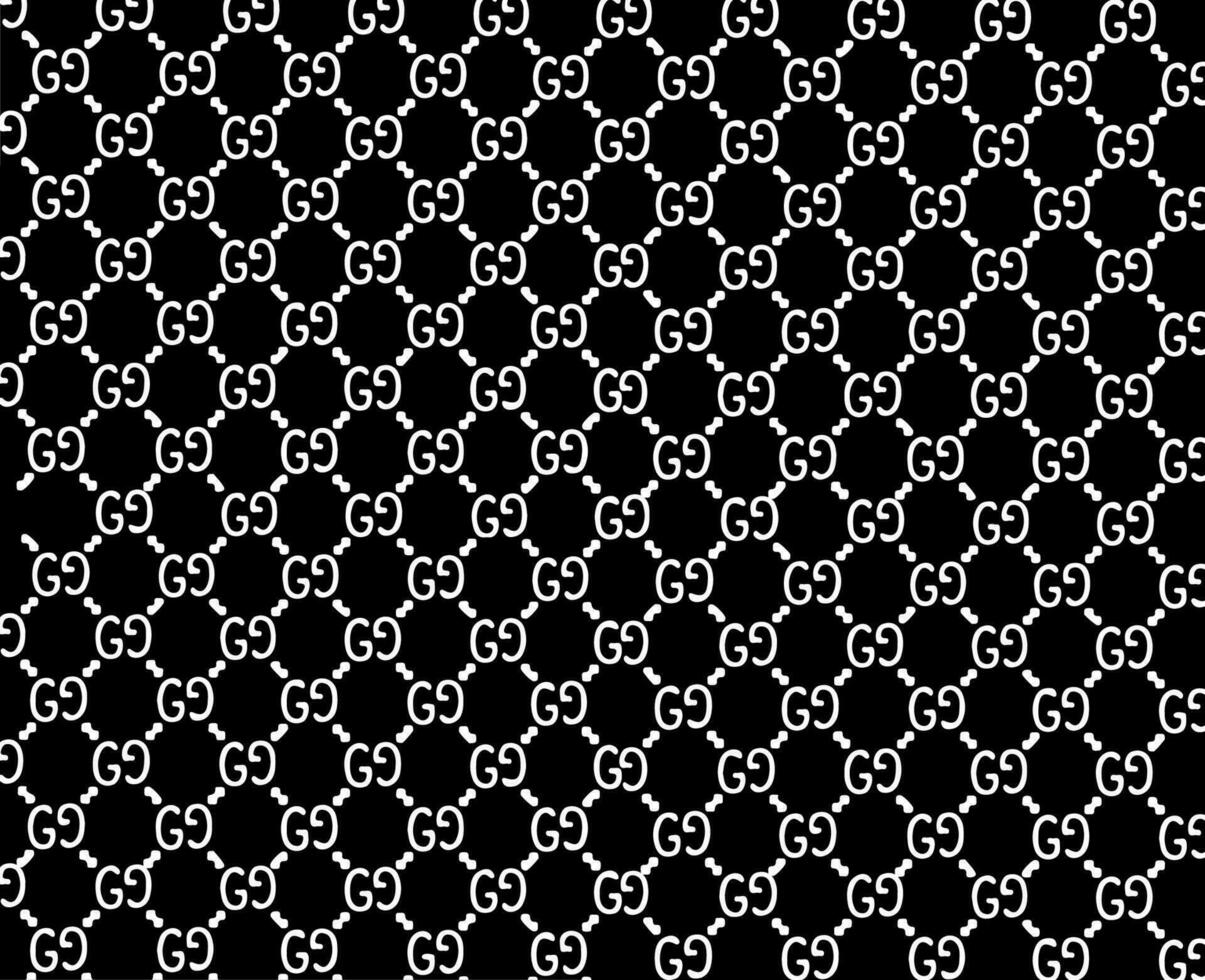The image displays a uniform, black-and-white repeating pattern on a black background. The design consists of hatch marks forming diamond shapes, reminiscent of a snakeskin or chain link fence. Each diamond's center point features symbols resembling an uppercase G and an inverted G, or the numbers 6 and 9. These symbols are consistently placed at every intersection where the lines bisect. The pattern is entirely symmetrical, evoking the design of a high-end fashion brand like Gucci. The graphic remains starkly monochromatic with no shading or color variations, creating a clean, flat appearance.